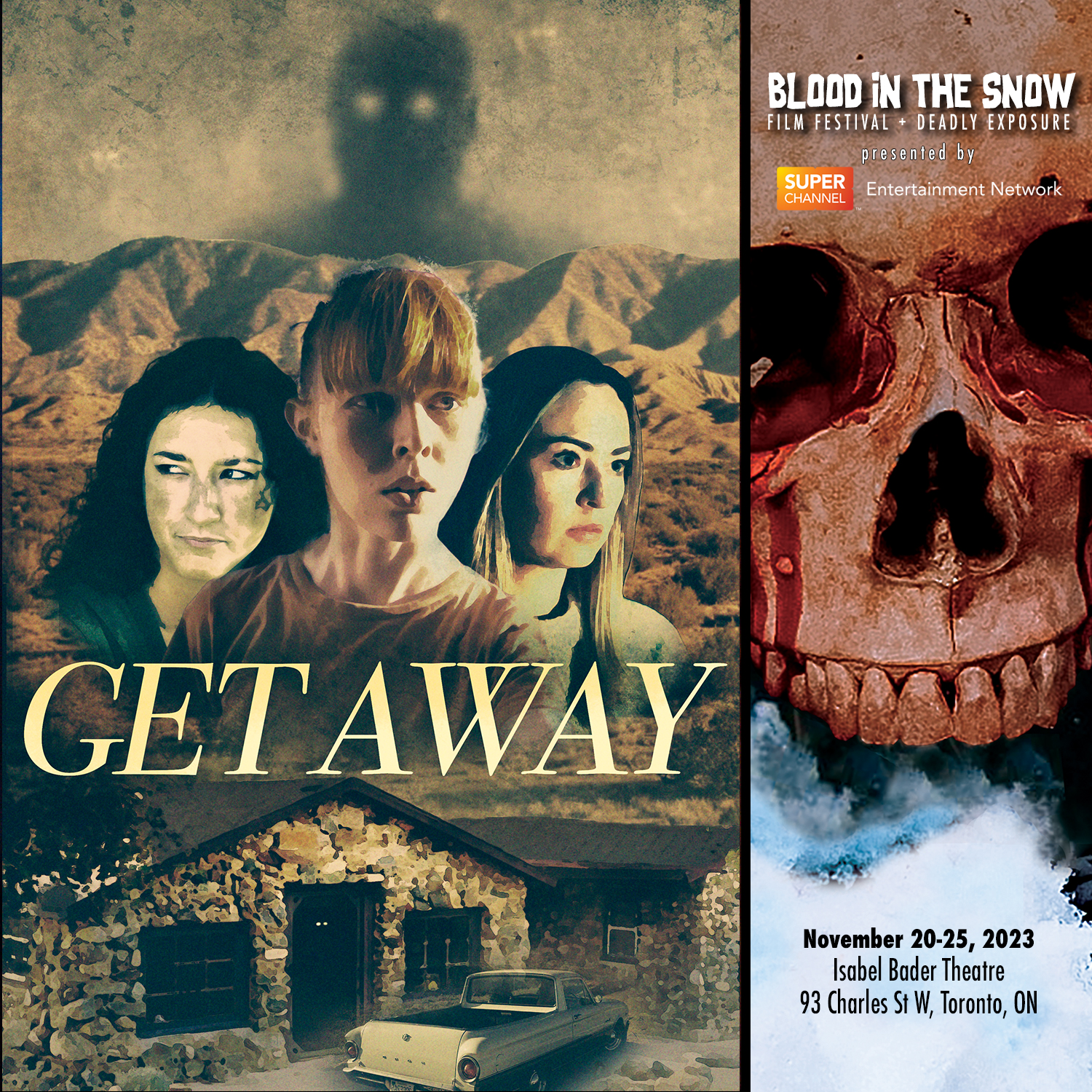The image depicts a dual-themed movie poster. Dominating the left side is a poster for a movie titled "Getaway," featuring three women positioned centrally. The woman on the left has dark hair, while the other two have blonde hair. They stand in front of a rugged mountain range, above which looms a shadowy, sinister figure with piercing white eyes. Below the women, there's an old brick house with a vintage car parked next to it, all set against a textured backdrop. On the right side of the image, there is information about the "Blood in the Snow Film Festival" and the film "Deadly Exposure," presented by Super Channel Entertainment Network. This section features a close-up of a red skull, seemingly shedding blood from its right eye onto what looks like white waves or snow. Detailed information about the event is provided: it takes place from November 20th to 25th, 2023, at the Isabel Bader Theatre, located at 93 Charles Street West, Toronto, Ontario.